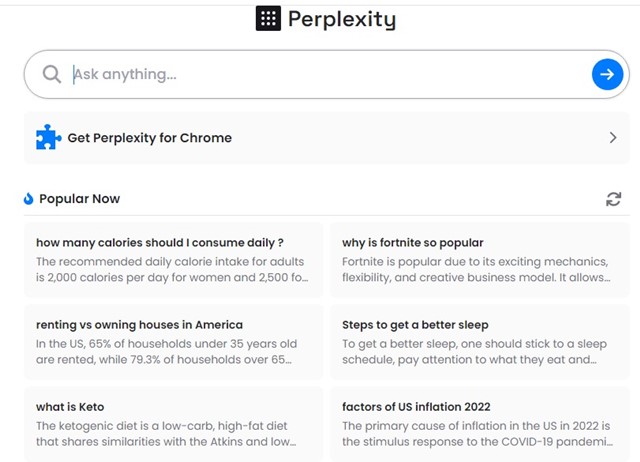The website features a sleek, minimalist design dominated by a black "Perplexity" header accompanied by a small black box containing three rows of tiny white dots. Below the header is a gray-outlined search bar with a gray magnifying glass icon and the prompt, "Ask anything." To the right of this search bar is a blue circle with a white arrow pointing to the right.

Beneath the main header section, the background transitions to a very light gray, highlighting a call-to-action banner in black text that reads, "Get Perplexity for Chrome." This banner includes a small blue puzzle piece icon and a right-pointing arrow. 

Further down, a "Popular Now" section showcases trending questions, each set within a gray-shaded banner and black lettering. 

1. "How many calories should I consume daily?" - The preview states: "The recommended daily caloric intake for adults is 2,000 calories per day for women, and 25..."
2. "Renting vs. owning homes in America" - The partial answer notes: "In the US, 65% of households under 35 years old are rented, while 79.3% of households over 65..."
3. "What is keto?" - Begins: "The ketogenic diet is a low-carb, high-fat diet that shares similarities with the Atkins and low..."
4. "Why is Fortnite so popular?" - Starts with: "Fortnite is popular due to its exciting mechanics, flexibility, and creative business model. It allows..."
5. "Steps to get better sleep" - Advises: "To get a better sleep, one should stick to a sleep schedule, pay attention to what they eat, and..."
6. "Factors of US inflation 2022" - States: "The primary cause of inflation in the US in 2022 is the stimulus response to the COVID-19 pandemic..."

Each question preview is designed for easy reading, with subtext in gray providing partial answers.